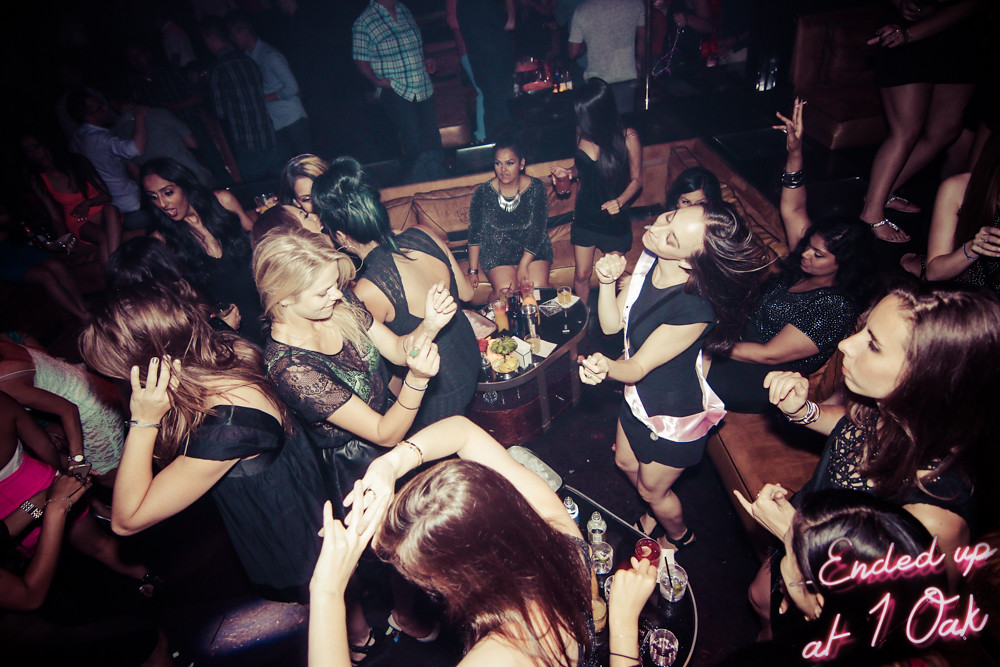The photograph captures a lively, crowded scene at a nightclub or lounge, with the ambiance primarily lit by the camera flash, casting a dim backdrop to the festivities. Dominating the center of the image are several women dressed in elegant black evening gowns, engaging in spirited dancing. One woman stands out prominently with a pink silk sash draped around her shoulder and hip, possibly indicating she’s the focal point of the celebration, such as a bachelorette party. To the back left, a brown leather corner couch accommodates numerous seated party-goers, while in front of them, a low, reflective, metal coffee table is strewn with an assortment of snacks and drink cups. There's a mix of seated and standing revelers, some of whom appear to be men clad in plaid shirts and jeans, lending an air of casual enjoyment as they indulge in drinks. In the lower right corner of the photo, the cursive pink text "ended up at one oak" is emblazoned in a neon-ish style, adding a stylish caption to the vibrant nightlife scene. The overall vibe is one of joyous celebration, enhanced by the chic attire and dynamic movement of the crowd.